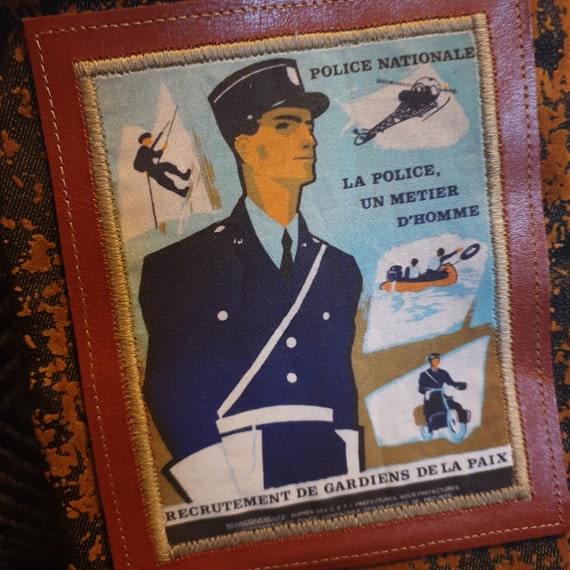This image depicts a meticulously detailed leather patch designed for the French Police Department, specifically the Police Nationale. The central figure on the patch is a young male police officer, proudly standing with his head held high, donned in a traditional French police uniform. His attire includes a dark blue cap, a dark blue suit with a white sash, white gloves, a white belt, a light blue shirt, and a dark tie.

Surrounding this central illustration are various vivid action scenes: an officer is shown rappelling down a mountain, another is riding a motorcycle, two individuals are depicted in an orange lifeboat with one throwing out a life preserver, and a black silhouetted helicopter is seen in flight, its blades clearly visible.

The patch's brown leather border is accented by a stitched white outline, adding to its distinguished appearance. The inscriptions are in French, with the top reading "Police Nationale" in bold black text, and the bottom featuring the phrase "Recrutement de Gardiens de la Paix," suggesting a focus on recruitment.

The patch exudes a sense of pride and duty, symbolizing the various challenging and dynamic roles within the police force. It's crafted from leather and is displayed on a backdrop resembling a brown and dark green tablecloth.